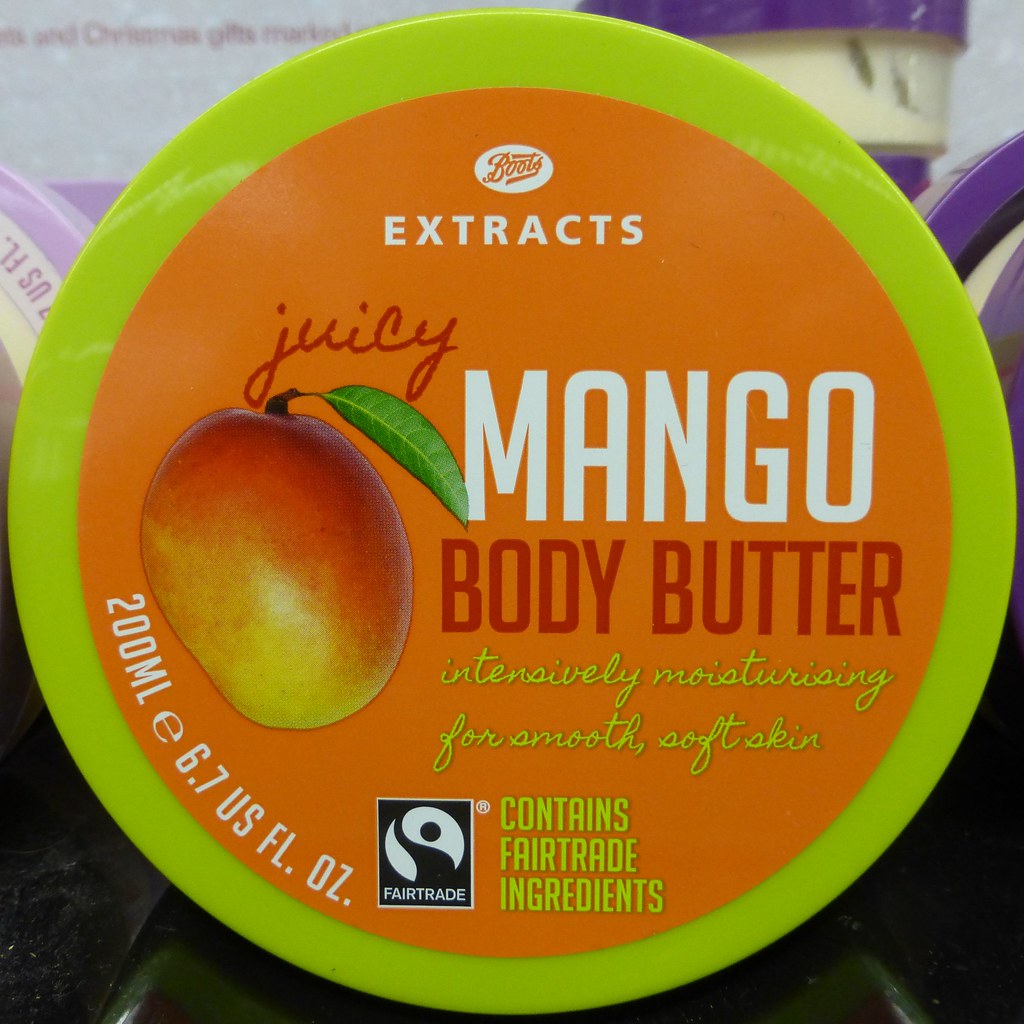The image shows a close-up of the top of a body butter package. The product is in a circular plastic container, which is neon yellow-green in color. A large orange sticker covers most of the container's lid. The sticker prominently features a white "Boots Extracts" logo at the top. Below the logo, on the left side, is a vivid photograph of a mango with a green leaf, accompanied by the word "Juicy" in red script above the fruit. To the right of the mango image, the product name "Mango Body Butter" is displayed with "Mango" in white text and "Body Butter" in red. Beneath this, in green script, it states, "Intensely Moisturizing for Smooth Soft Skin." At the bottom of the label, it reads "Contains Fair Trade Ingredients" in green text, with a black and white Fair Trade logo to the left. Additionally, the label includes the product volume, "200 milliliters, 6.7 US fluid ounces," in white text on the lower left side.